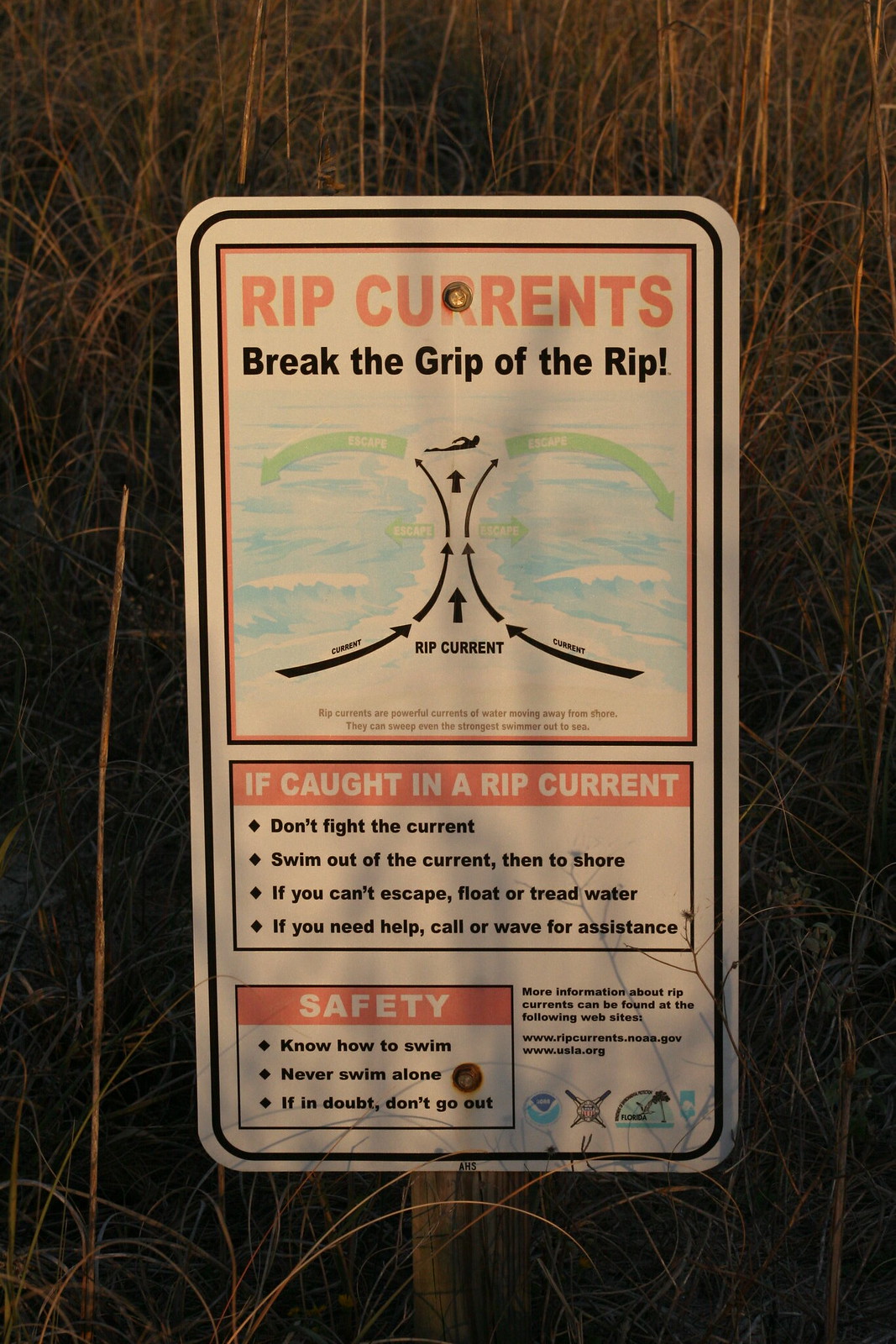The image showcases a weathered, wooden signpost standing amidst tall, dry brown and yellow grass. Mounted on the post is a vertical white rectangle sign with a narrow black border. The sign is slightly faded from the sun and divided into three distinct sections outlined with small black borders. 

At the top of the sign, within a red-bordered rectangle, bold red capital letters announce "RIP CURRENTS" followed by the phrase "Break the Grip of the Rip" in black text. Below this header lies an instructional diagram illustrating the behavior of rip currents, including directional arrows and a figure swimming parallel to the shore to escape the current.

The middle section features a header with a red border titled "If Caught in a Rip Current." Beneath this, in bullet points, are four crucial safety instructions: 
1. Don't fight the current.
2. Swim out of the current, then to shore.
3. If you can't escape, float or tread water.
4. If you need help, call or wave for assistance.

The final section, labeled "Safety," contains three important safety reminders in bulleted format:
- Know how to swim.
- Never swim alone.
- If in doubt, don't go out.

Adjacent to these instructions, additional information points visitors to resources about rip currents, listed as URLs near the bottom right corner along with some logos. The detailed and instructive sign aims to educate on rip current safety within the natural, grassy setting.